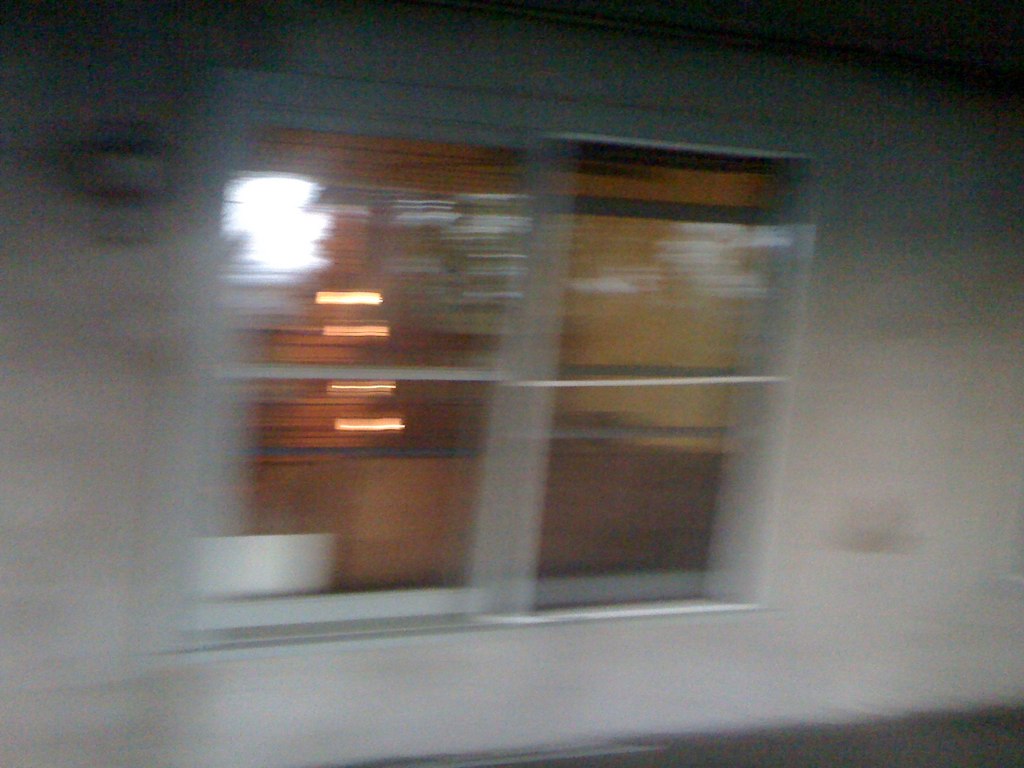This photograph, albeit blurry, depicts a window with two panes. The image primarily consists of the window's outline against a predominantly white background, hinting at its potential for movement, particularly the lower pane. Reflections play across the glass, interspersed with some darker areas that obscure clear identification of the interior contents. Therefore, this scene likely captures the view of a room from the outside. Within the reflections, there are various shades of brown and an orangey-red light, divided into four rectangular segments. Additionally, a white object in the window's bottom left corner, possibly the top of a chair or a flower pot, adds an element of intrigue to the indistinct scene.